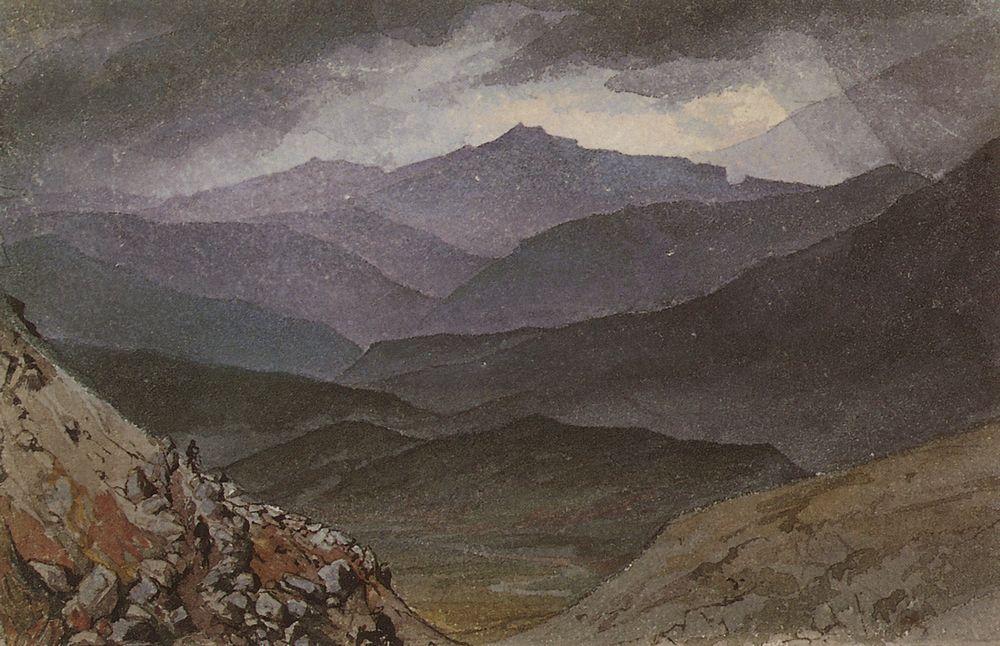The image depicts a striking, modern scene of a mountain valley at either sunrise or sunset, characterized by several layers of mountains that extend across two-thirds of the frame. The mountains, painted in deep purples, dark grays, and nearly black hues, create a sense of depth and dimension, enhanced by the foreground details like rocky cliffs and tan boulders. The sky above is dramatic, with dark gray clouds punctuated by lighter patches, adding to the overall moody atmosphere. On the left side, a path winds through the mountains, where a figure is seen walking away from the viewer, and another figure stands at the edge, gazing out over the expansive, lush green valley below. To the right, a smooth, brown mountainside contrasts with the detailed granite rocks that dot the foothills, leading the eye toward the distant horizon where the mountain range unfolds beneath the brooding sky.